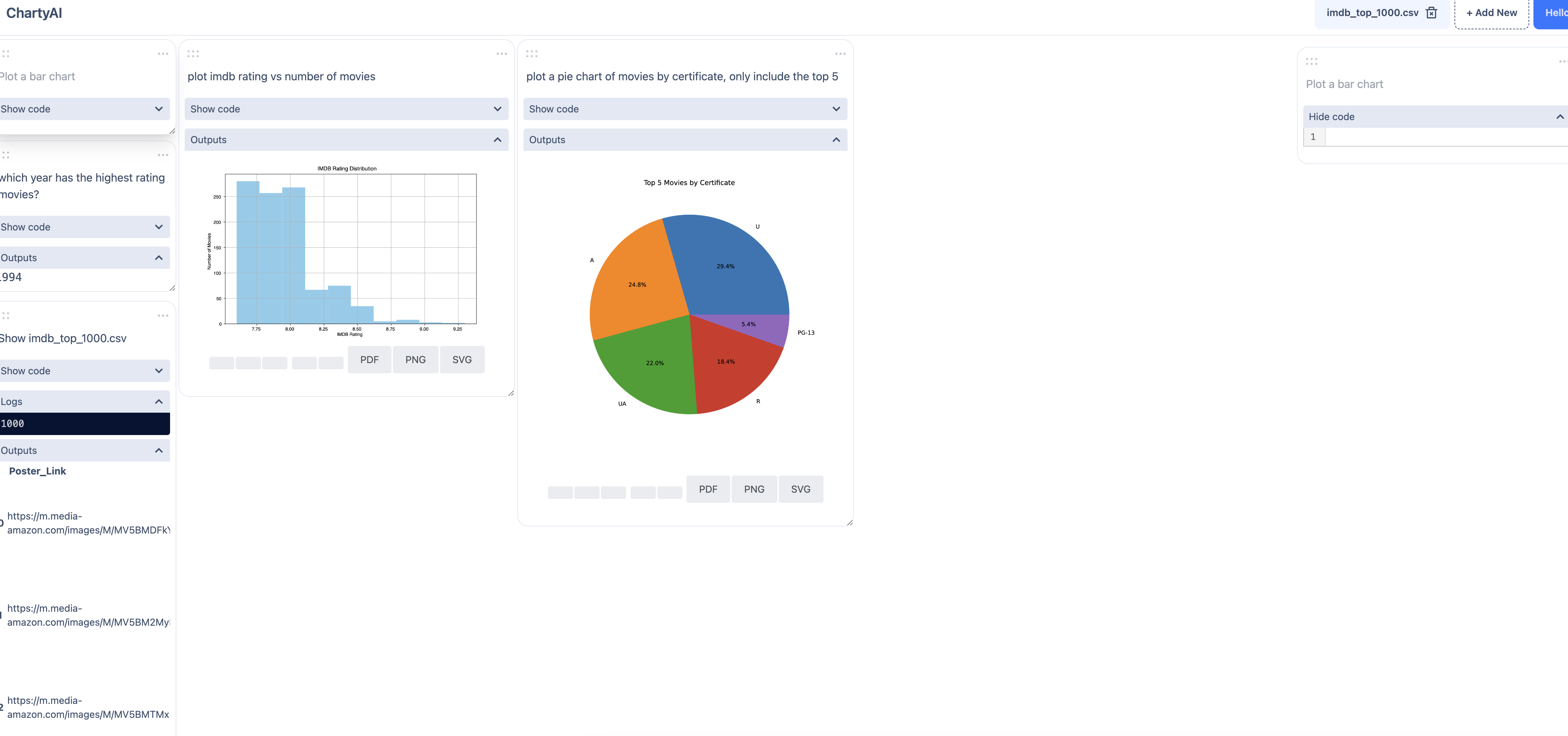The image depicts a predominantly white screen, matching the white background of the application in question. In the top left corner, the text "CHARTYAI" is displayed in very small letters, with only the 'C' and 'A-I' capitalized. On the top right, there is a white button outlined with dotted gray lines, labeled "INSIDE" in gray, alongside a plus sign and the phrase "ADD NEW" also in gray. Adjacent to it is a blue button, containing the word "HELLO" followed by an exclamation point in white text. Beneath these buttons is a faint gray horizontal line running across the screen, with the majority of the screen remaining empty. The image exclusively uses the colors black, white, gray, and blue, with minimal information taking up just a fraction of the largely blank white space.